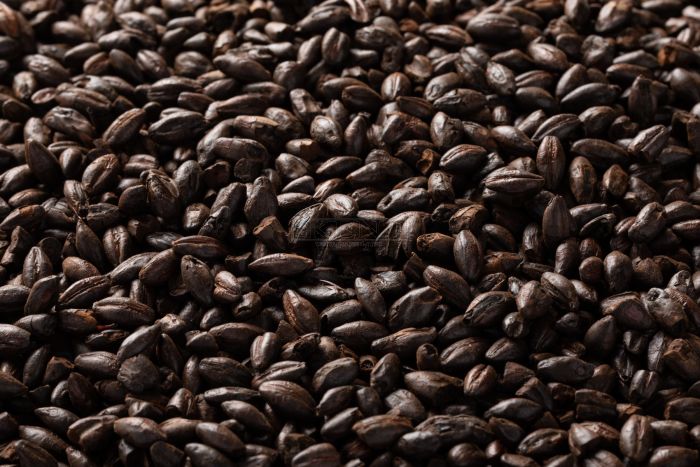The photograph showcases an extensive and detailed close-up of dark roasted coffee beans, filling the entire frame. The coffee beans, varying in shades from dark brown to nearly black, cover the entire image without revealing any background or context, making it seem as though one is peering into a deep collection or perhaps a container brimming with these aromatic seeds. The beans exhibit their characteristic oval shapes with a few displaying subtle reflections of light, adding texture to the overall composition. While most of the beans are sharply in focus, some toward the upper portion of the image are slightly blurred, creating a natural depth. This meticulous capture emphasizes the rich, dark hues of what are unmistakably roast coffee beans.